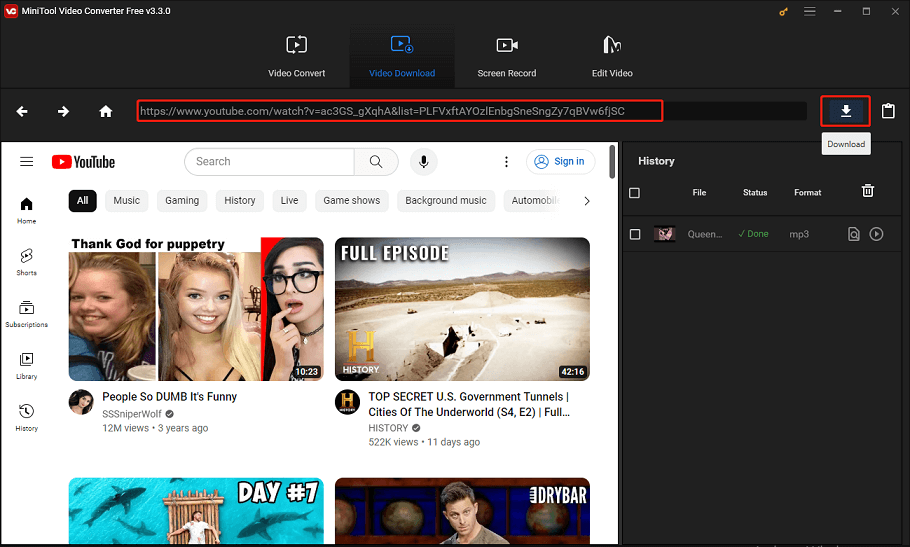This is a detailed screenshot of a YouTube page with various options at the top, including "Video Convert," "Video Download," "Screen Record," and "Edit the Video." The "Video Download" option is currently selected, indicated by a blue checkmark. The search bar shows a long URL, starting with "youtube.com/watch" followed by numerous characters.

The first visible video on the screen is titled "Thank God for Puppetry: People So Dumb, It's Funny," which accumulated 12 million views over three years. The next video is a full episode from the History Channel titled "Top Secret United States Government Tunnels: Cities of the Underworld," specifically Season 4, Episode 2. This video is 42 minutes long and received 522,000 views in the past 11 days.

Below these, only the top portions of two more videos are visible. One appears to be titled "Day Number Seven," featuring an image of a man on a small floating log raft surrounded by fish and sharks. The other partially visible video is from "Dry Bar," showing just the top of a man's head.